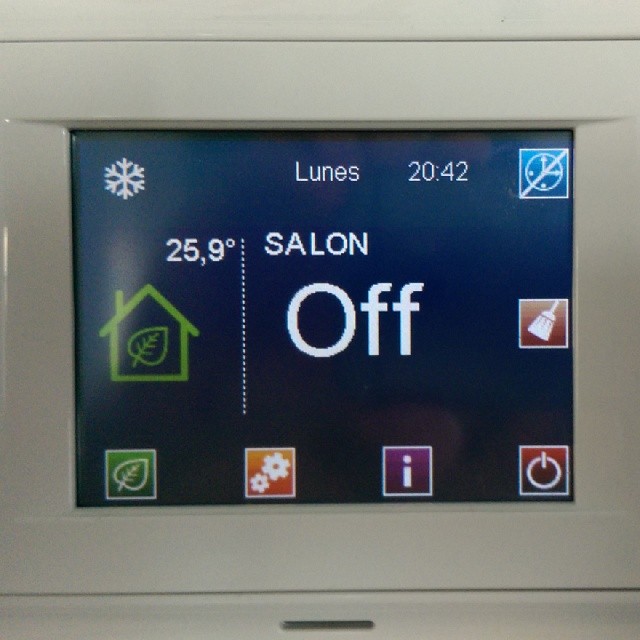This image depicts a digital thermostat, rendered with a graphic or possibly an extreme close-up photograph technique. The thermostat itself is an off-white or beige color and is cropped closely so that the edges are not visible, focusing the viewer's attention on the central digital display.

The display is rectangular, being slightly longer in length than in width. In the upper left-hand corner of the display, there is a white snowflake icon. Just below it, the screen displays "LUNAS" in white lettering, indicating that it is Monday in Spanish. The time shown is 20:42. To the right of these indicators, there is a blue square containing a clock icon with a line through it, suggesting the time setting feature is disabled.

At the center of the display, the label "SALON" is prominently featured in capital letters, likely indicating the thermostat is placed in or controls the living area. Directly below this, in larger white letters, the word "OFF" is displayed, indicating the thermostat is currently turned off.

The bottom section of the display contains several colored square icons: 
- In the lower left-hand corner, a green square with a leaf represents an eco or energy-saving mode.
- Next to the green square, an orange square with gears signifies the settings menu.
- To the immediate right, a purple square with an eye icon suggests an information or status check feature.
- Completing the icon row, the lower right-hand corner features a standard power button, depicted in red and black with the familiar on/off symbol (a circle with a vertical line).

Overall, the image provides a detailed view of the thermostat's display and various settings, offering a clear and thoughtfully designed interface for temperature control.